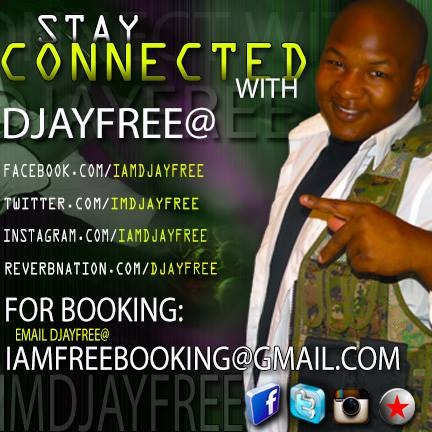This image appears to be a promotional banner ad or social media card advertising a DJ known as DJ Free. The photograph features a young, smiling African-American male DJ with a shaved head, who is striking a dynamic pose by throwing a sideways peace sign. He is dressed in a camo vest over a white long-sleeved shirt which itself is layered over a black t-shirt. The background is a dark green and purple splotchy pattern, enhancing the vibrant and energetic feel of the ad.

Text on the left side of the ad reads: "Stay connected with DJ Free at facebook.com/imdjayfree, twitter.com/imdjayfree, instagram.com/imdjayfree, reverbnation.com/djayfree." Directly beneath, it states, "For booking, email djayfree at imfreebooking@gmail.com." Additionally, the bottom right corner features logos for Facebook, Twitter, Instagram, and a silver circle with a red star, likely representing ReverbNation.